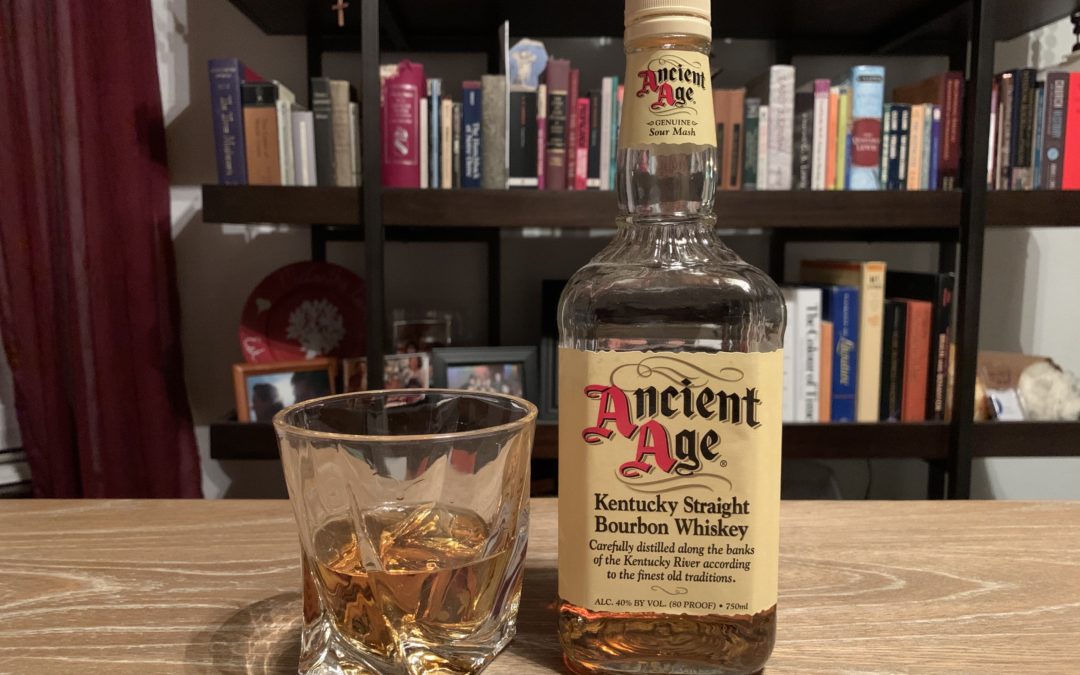The image, taken indoors, showcases a brown wooden table at the bottom. On the left side of the table rests a whiskey glass, half-filled with a golden liquid. Beside the glass, there is a nearly half-empty bottle of Ancient Age Kentucky Straight Bourbon Whiskey. The bottle’s label features the words "Ancient Age" with the two A’s in red and the other letters in black. Beneath the label, it specifies, "carefully distilled along the banks of the Kentucky River according to the finest old traditions," and notes the alcohol content as 40% by volume (80 proof) in a 750-milliliter bottle. 

In the background, there is a multi-tiered bookshelf. The lower tier holds photos with frames of various colors, some books, and a few knickknacks, including a red plate adorned with a heart and possibly a tree or plant design. The upper tier is completely filled with books of various colors, stretching from one side to the other. The bookshelf itself is brown-framed and appears to be supported by metal. Additionally, a burgundy curtain is seen in the back, adding warmth to the interior setting. The overall arrangement places the bottle of whiskey as the central focus, with the glass nearby, both grounded by the simple yet detailed surroundings.